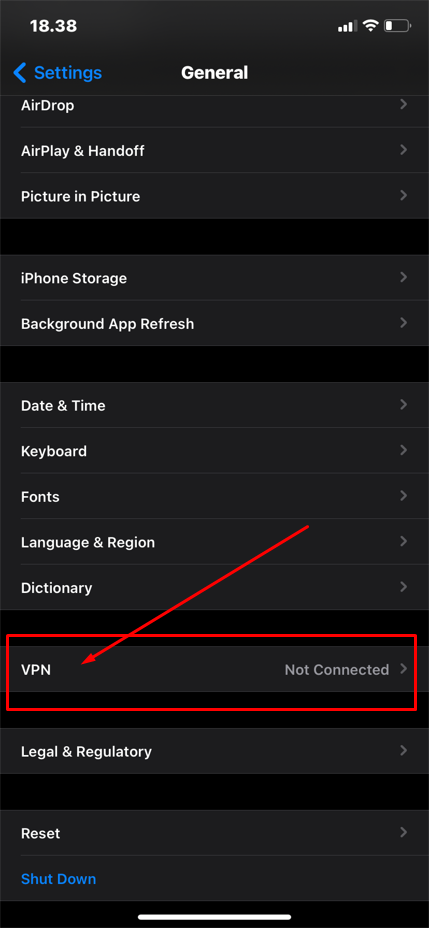In this screenshot of a mobile application, the layout is predominantly black with various shades of gray and blue elements. At the top, there's a dark gray header accented by white icons. On the left side of the header, a blue arrow points left, followed by the blue text "Settings." Centered at the bottom of the header is the white text "General," beneath which runs a thin medium gray line spanning the page's width.

Below this, three rows of white text are displayed, each separated by similar gray lines. On the right side of each row is a light gray arrow pointing right. The text in these rows is, from top to bottom: "AirDrop," "AirPlay & Handoff," and "Picture in Picture."

Further down, a black rectangle spans the screen's width, followed by two more rows with white text and light gray arrows. These rows are labeled, from top to bottom: "iPhone Storage" and "Background App Refresh."

Another black rectangle appears beneath these, followed by five more rows of similarly formatted information. These rows are labeled, from top to bottom: "Date & Time," "Keyboard," "Fonts," "Language & Region," and "Dictionary."

Yet another black rectangle appears, followed by a single row with a dark gray background. This row labels "VPN" on the left, with the smaller light gray text "Not Connected" on the right, and another light gray arrow pointing right.

Overlaid on the screen is a red rectangular outline, with a red arrow coming down at a 45-degree angle from the top right, pointing toward the "VPN" text.

The final element in the screenshot, after another black rectangle, is a single row labeled "Legal & Regulatory."